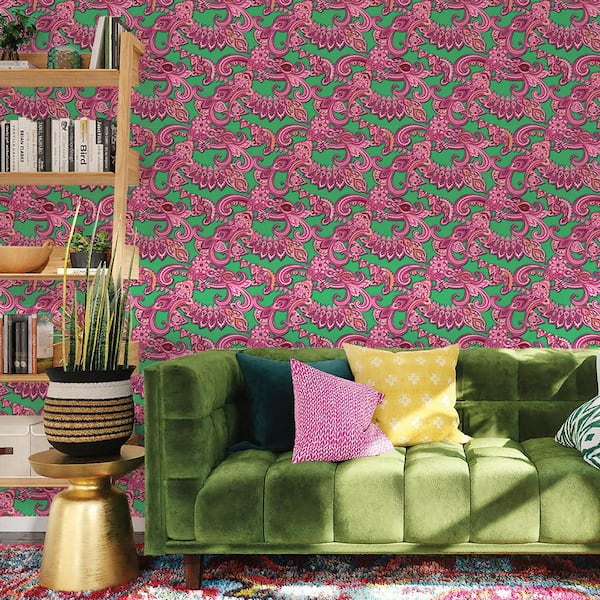In this vibrant image of a living room, the retro 70s-style wallpaper stands out with its green backdrop adorned with intricate pink and purple patterns. Dominating the scene is a plush green couch bathed in sunlight, which spans from the center to the right edge of the image. The couch is decorated with three throw pillows clustered on the left corner, in hues of pink, yellow, and blue, alongside another pillow on the right in green and white.

To the left of the couch, a small golden table adds a touch of elegance, topped with a striped pot housing a lush green plant. Behind it, a wooden bookshelf stretches off the image with multiple shelves filled with various items. The second shelf holds what appears to be CDs, while a brown bowl and another pot sit on the third shelf. The fourth shelf showcases a collection of books, with additional books or objects and a small plant occupying the topmost shelf.

The room is anchored by a multicolored carpet that features a seemingly random design incorporating shades of red, blue, yellow, and white, enhancing the eclectic and cozy atmosphere of the space.